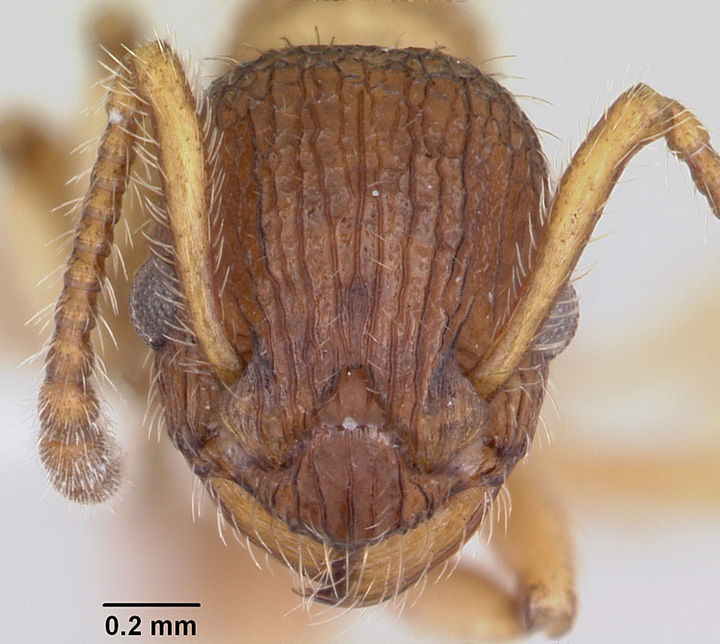This image showcases an extreme close-up of a very small insect, likely an ant, dominated by its intricate head and upper body. The frame features the insect's head, which occupies most of the space and measures approximately 2 millimeters in length and 1 to 1.2 millimeters in width. The insect's head is dark brown near the eyes and mouth area, lightening slightly around the rest of its head. Prominently displayed are its two compound eyes, which are gray in color, and situated on either side of its head. The head also features two antennae that extend outward and then bend downward, covered in fine, white hairs. Just under the head, there's a small line marked "0.2 millimeters" for scale, emphasizing the insect's minute size. The remaining parts of the body, which appear slightly blurred in the background, hint at a compact and oval-shaped form, similar to a walnut in shape. The details like the fine hairs, compound eyes, and antennae are meticulously captured, providing a stunning macro perspective of this tiny creature.